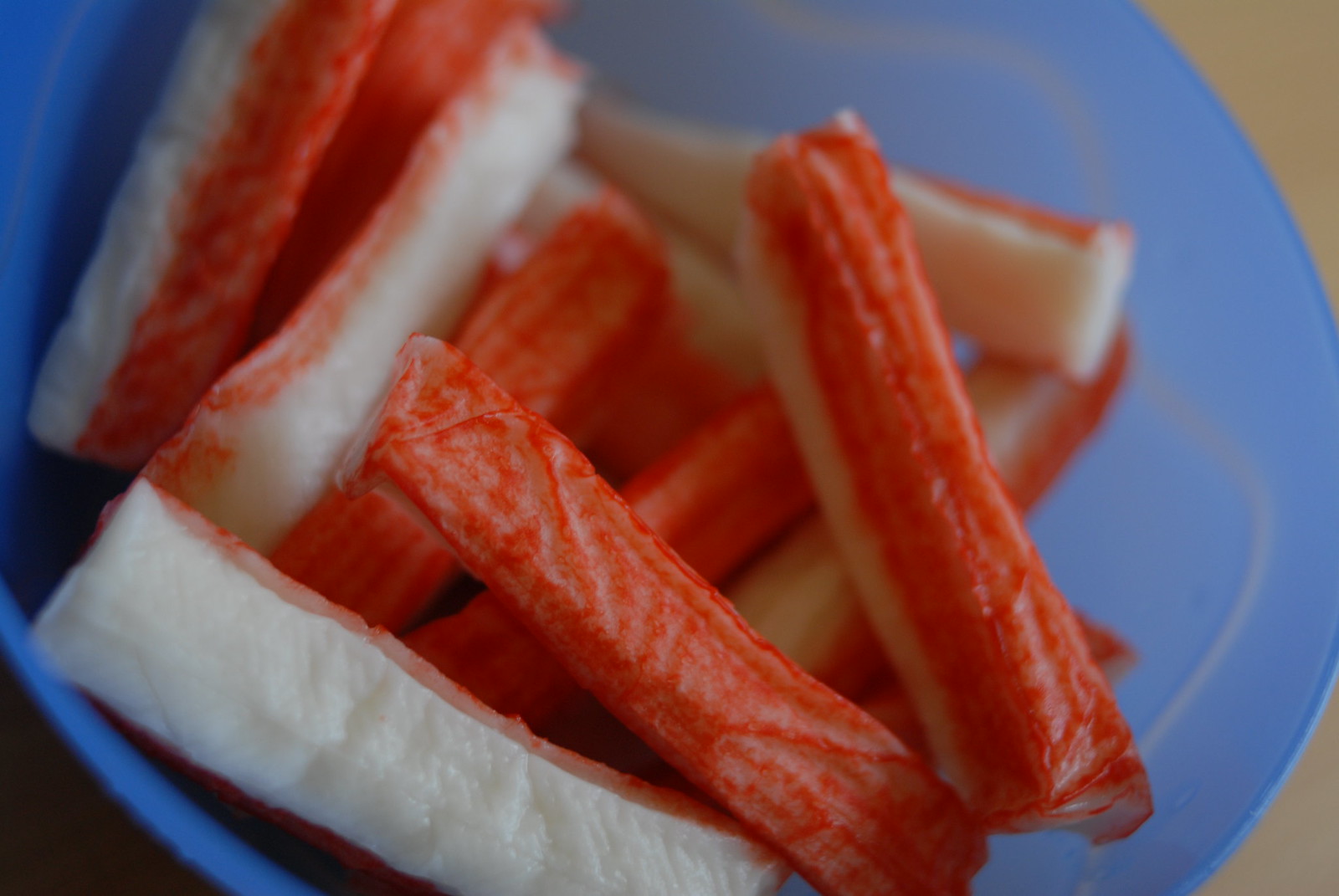The image depicts a close-up of a blue plate, possibly made of plastic, sitting on a tan-colored surface. The plate holds a substantial amount of imitation crab meat sticks, approximately 15 to 20 pieces. These sticks, which are long, rectangular, and skinny, are characterized by their white bottom half and reddish-orange top half, offering a textured appearance. They are neatly stacked, primarily in the front and center of the plate, resembling a pile of matchsticks. The arrangement includes three sticks leaning diagonally in the foreground, while the rest are either aligned horizontally or stacked diagonally in the opposite direction. The right edge of the plate catches some light, giving it a slight silvery glimmer. The overall presentation suggests that the imitation crab sticks might be crunchy and chewy.